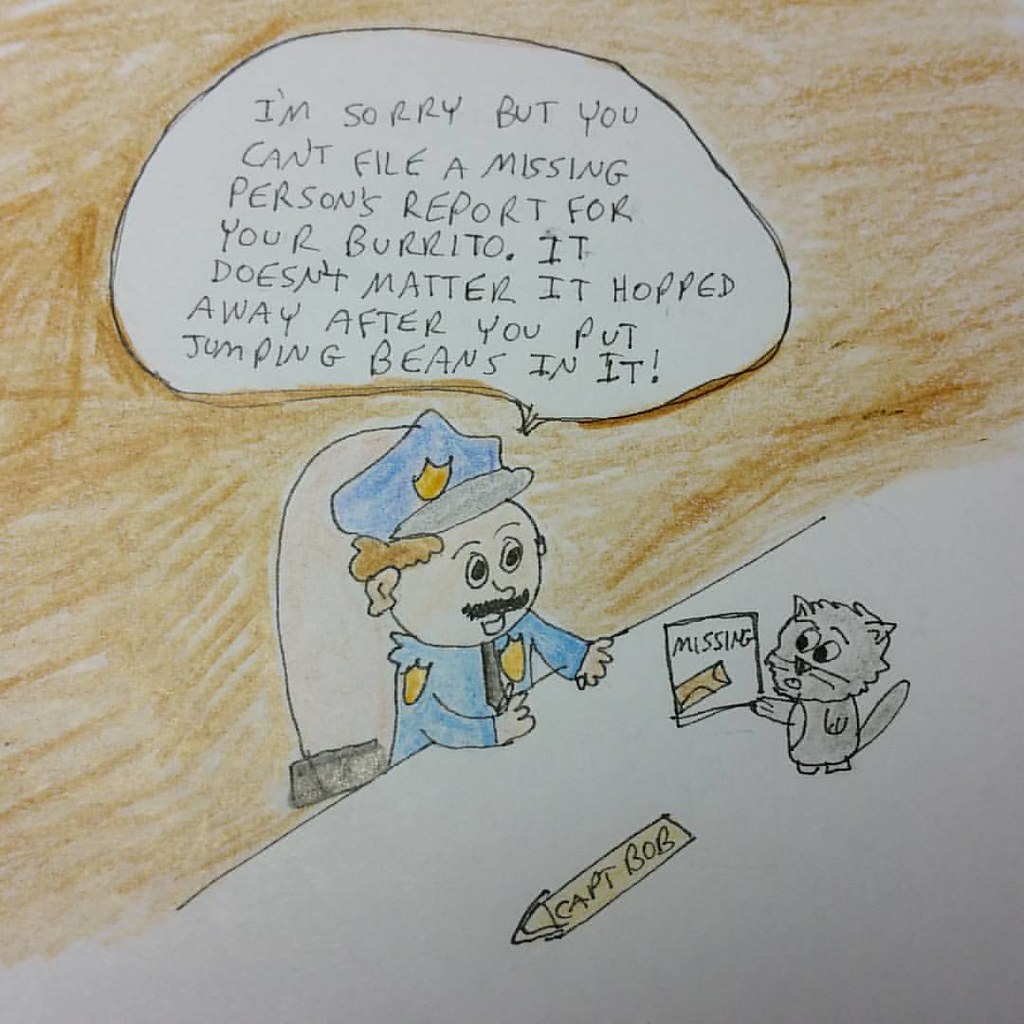In this whimsical, cartoon-style drawing, a police officer with brown hair, a black mustache, and a blue uniform adorned with yellow badges is sitting behind an implied white counter. The name "Captain Bob" is displayed on a yellow nameplate on the desk. Across from him stands a small, gray cat, holding a piece of paper with the word "missing" written on it. The officer is featured in a speech bubble surrounded by a brown area, saying, "I'm sorry, but you can't file a missing person's report for your burrito. It doesn't matter; it hopped away after you put jumping beans in it."